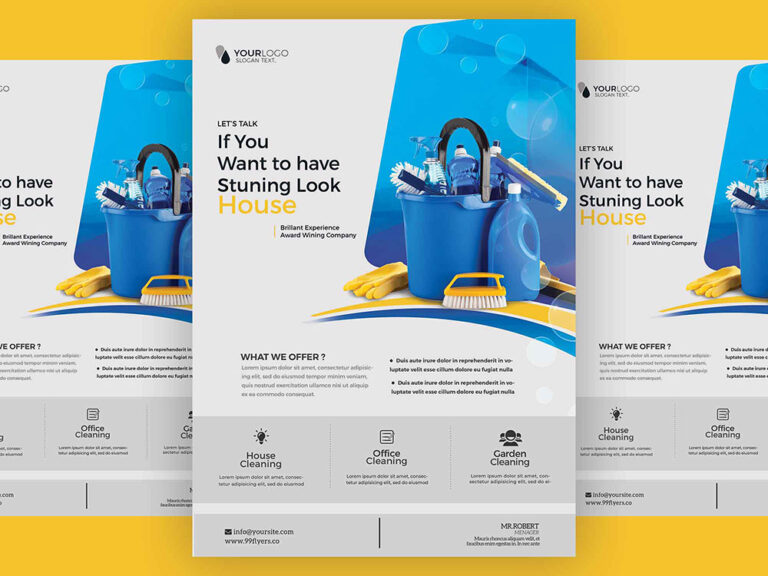The image showcases a website advertisement prominently displayed in the center of a rectangular poster with a light gray background. The poster is flanked by two similar, smaller posters on either side against a yellow backdrop, hinting at a cohesive promotional display. The central advertisement features a distinctive logo reading "Your Logo" followed by slogan text, suggesting it may be a website aimed at creating custom slogans. 

At the top right corner of the poster is an image of a blue bucket filled with various cleaning items. Among these items are a blue plastic bottle resembling a laundry detergent bottle with a white cap and handle, a yellow scrubbing brush with a yellow handle, and a pair of yellow gloves. 

Adjacent to the bucket, there are additional cleaning supplies, including brushes and bottles. On the left side of the poster, bold white text reads, "Let's talk if you want to have a stunning-looking house," with further details about the product provided below. This thorough arrangement, combined with the mirrored smaller posters, creates a visually appealing and informative advertisement.